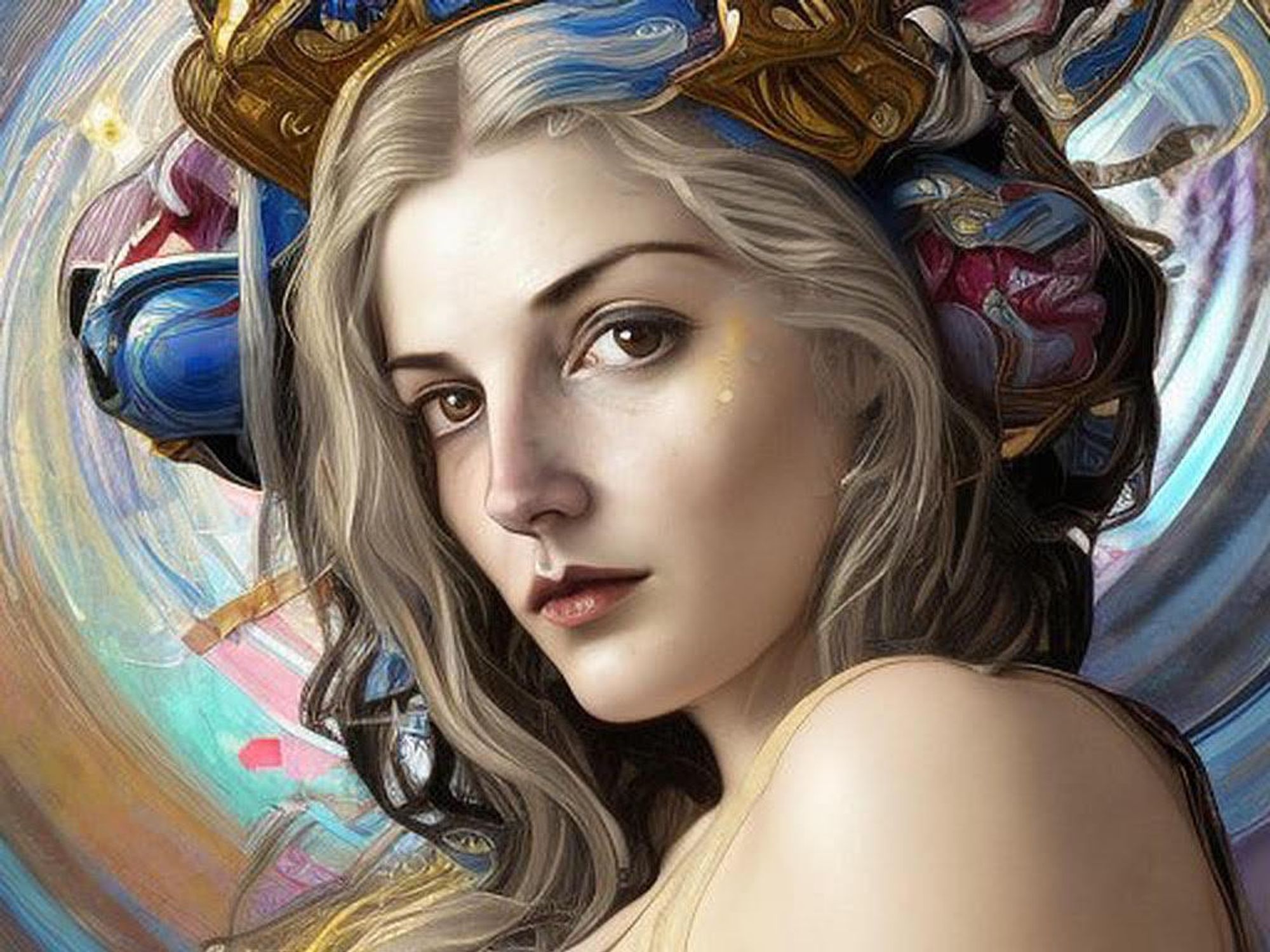The image is an intricately detailed painting of a strikingly beautiful woman, centrally positioned and gazing directly at the viewer. She is depicted from just below the shoulders upwards, clothed in a yellowish outfit with visible shoulder straps. Her face, meticulously painted with thin black eyebrows, prominent cheekbones adorned with a hint of blush, and red lips, suggests classical beauty. Her long, blonde hair, parted down the middle, features subtle brown tips and a hint of blue dye. Adorning her head is an ornate headgear, embellished with intricate patterns in blue, red, and gold, reminiscent of both fantasy and historical aesthetics. The background is a swirling tapestry of blue, orange, and pink hues, contributing to the painting's abstract, almost futuristic ambiance.